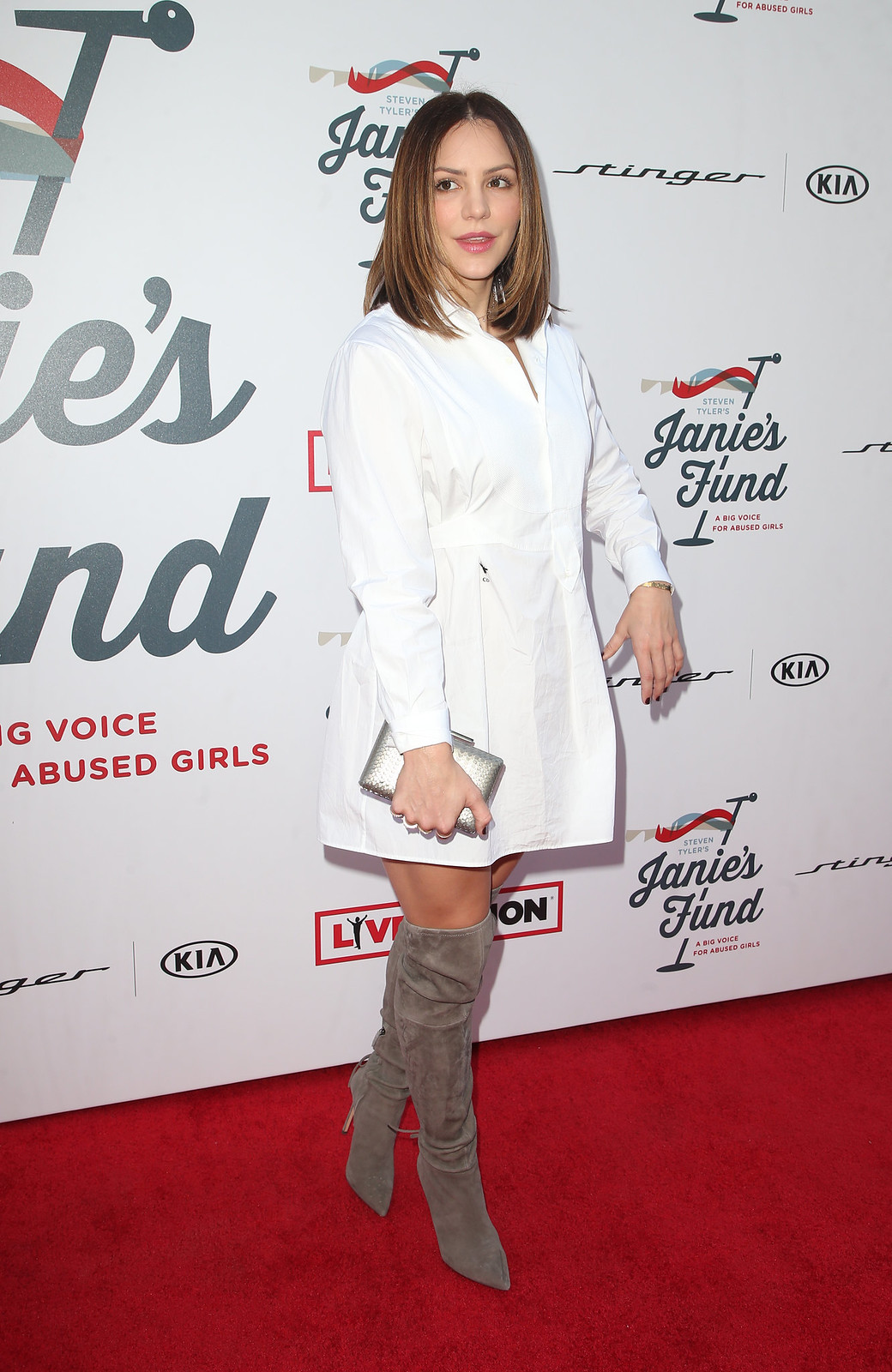In this photograph, a blonde-haired woman, with straight hair parted in the middle, is striking a pose on the red carpet at a charity event called "Janie's Fund: A Voice for Abused Girls," highlighting a microphone logo. She is wearing a stylish white long-sleeve jacket dress that is cinched at the waist and falls to her thighs. Her ensemble is completed with over-the-knee, tan-colored suede boots with high heels and a silver clutch bag in her right hand. Behind her, a backdrop showcases the sponsors of the event, including Kia and Live Nation, with several logos prominently displayed. The woman is looking directly at the camera, capturing the essence of this glamorous yet impactful occasion.